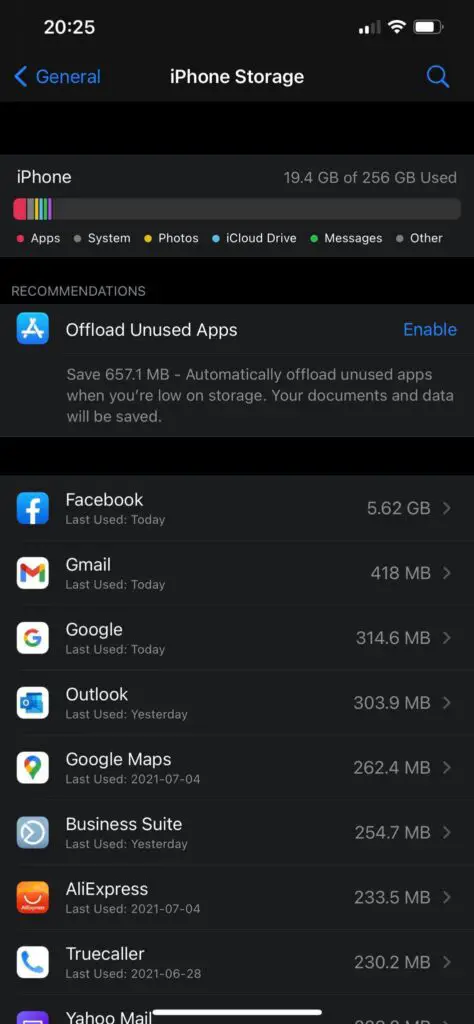This image is a detailed screenshot of an iPhone storage menu displayed on a black background. The interface primarily uses white and grey text, with various app symbols in color. 

At the very top-left corner, the current time is shown as "20:25". On the top-right corner, there are icons for signal strength, WiFi strength, and battery level. 

Below this header, on the left side, there's a blue label "General" with an arrow pointing to the left, indicating a navigation option to go back to the previous menu. On the top-right side, a magnifying glass icon represents the search function.

Centered prominently in white text, the menu title "iPhone Storage" is displayed. Directly underneath, there's a detailed usage bar. On the left, it reads "iPhone," while on the right, it specifies "19.4GB of 256GB used" in pale grey text. The bar is color-keyed to indicate different storage categories, such as Apps, System, Photos, iCloud Drive, Messages, and Other, each represented by distinct colors like red, yellow, blue, and green. This bar visually depicts the storage space utilized by each category.

Under the usage bar, a "Recommendations" section suggests to "Offload Unused Apps," providing an option to enable this feature along with the amount of space that could be saved.

Below the recommendations, the largest space-consuming apps are listed in descending order. Each app name appears in white text along with its corresponding icon to the left. Below each app name is additional information in pale grey, and on the far right, the storage used by each app is displayed in gigabytes, accompanied by a right-facing arrow. The list starts with Facebook, followed by Gmail, Google, Outlook, Google Maps, Business Suite, AliExpress, Truecaller, and Yahoo Mail.